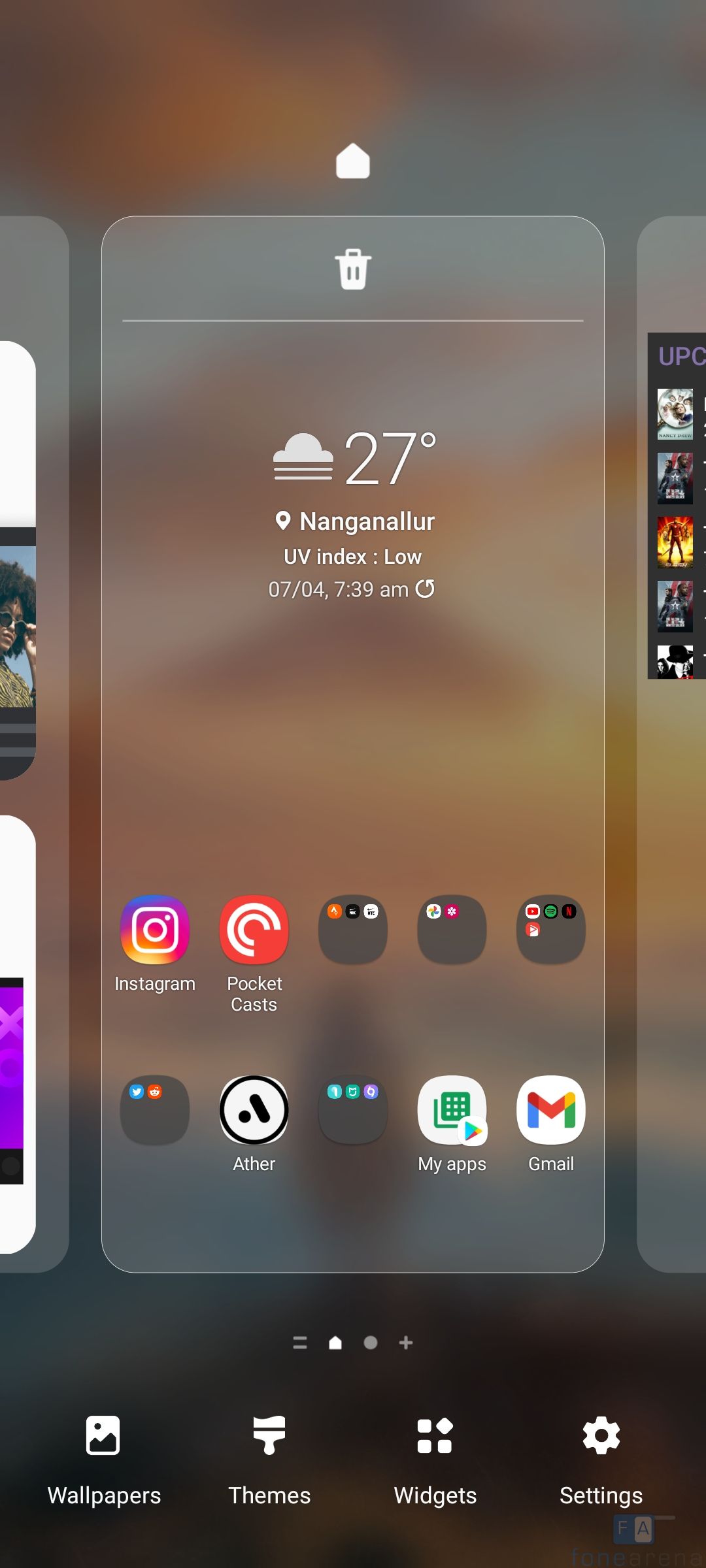This portrait-oriented photo captures a cell phone screen and is roughly three times taller than it is wide. The image focuses on the phone's interface, featuring multiple clear rectangular icons with curved edges set against a blurry background.

In the center, a prominent bubble is entirely visible, while two partial bubbles are seen on the left and right edges of the screen. The center bubble displays various widgets and app icons. At the top, there is a garbage can icon centered with a white border beneath it. Below this, a weather widget displays a cloud icon and reads "27°C," accompanied by a location marker tagged "Nangaralur." Additional information includes "UV index low" and the alphanumeric sequence "704," likely indicating the date. The time is shown as "7:39 AM," along with a refresh button.

Beneath the weather widget, a row of app icons begins with "Instagram" followed by "Pocket Casts." Next are three icons bundled inside a gray bubble, followed by another similar bundle with two icons. A noticeable white circle with the label "Ather" contains black elements inside it. Following this are icons for "My Apps" and "Gmail."

Overall, this photo showcases a personalized arrangement on someone's cell phone screen, highlighting both utility and aesthetic elements.